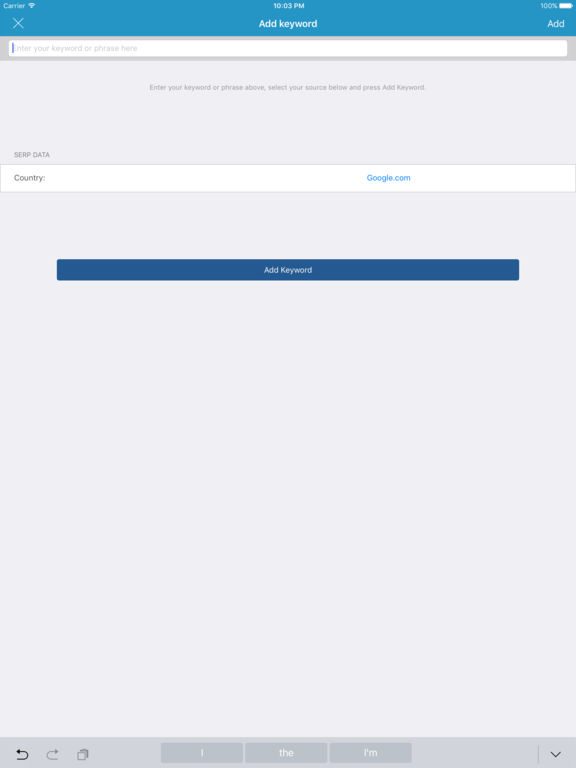This image showcases a detailed screenshot of a website interface. At the very top, there is a blue menu bar. On the top left corner, it displays the word "Carrier" accompanied by a Wi-Fi icon. Just beneath this, there's a white 'X' symbol. Centrally positioned within this bar, the time is displayed as 10:03 p.m., and towards the right, it indicates "100% battery" along with the word "Add".

Below this top menu bar is a search bar enclosed in a gray border, which features the placeholder text: "Enter your keyword or phrase here." Directly under this search bar, instructional text reads: "Enter your keyword or phrase above, select your source below, and press add keyword."

Following this instruction, there's another white box labeled "Country" with a dropdown menu, defaulting to "google.com" alongside it. Below this, in a blue box, there's an option labeled "Add Keyword."

The background of the main screen is largely gray. Towards the bottom section of the page, there is a darker gray menu bar featuring a reverse arrow on one side, a forward arrow on the other, and a copy icon. Additionally, there are three buttons labeled "I", "the", and "I'm" in smaller, darker gray boxes. Finally, in the bottom-right corner, there is a dropdown menu.